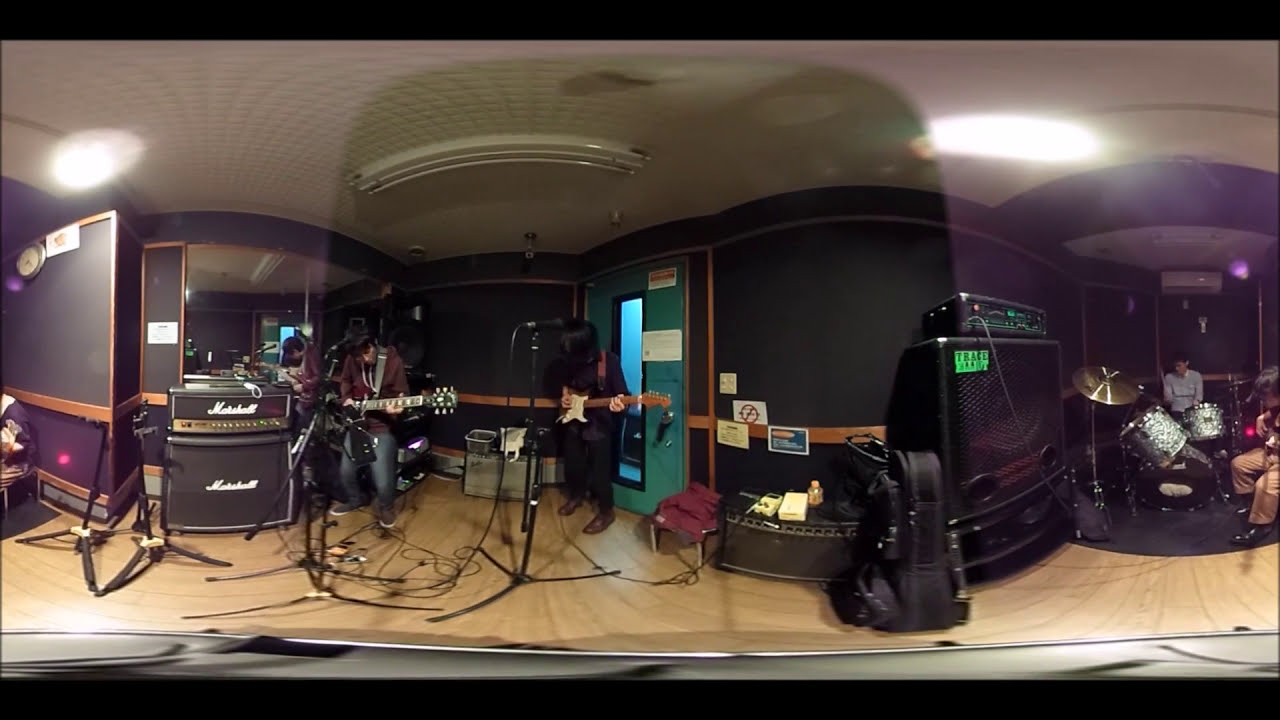The image captures the interior of a music studio, viewed through a distorted camera lens that bends straight edges into curves. On the left side of the room, a person with shoulder-length black hair, clad in a maroon long-sleeve shirt and blue jeans, holds a black guitar that faces right. Their head is bowed, one hand gripping the guitar's neck while the other rests on its body. Adjacent to them stands a black amplifier labeled "Marshall" in white letters, featuring a copper-colored instrument panel with knobs between the top and bottom sections. Nearby on the right, another person is seated at a silver sparkle drum set, partially obscured by a gold cymbal slightly to their left. 

Centered in the background, an open door emits a soft blue light, contrasting against a green-colored door frame. The room's wooden floor, scattered with musical equipment like carrying cases and speakers, adds a warm tone. Purple walls flank the sides with green in the middle, accented by bright white ceiling lights, one circular on the left and an oval-shaped one on the right. The scene is bathed in hues of black, tan, white, pink, purple, gray, silver, green, and light blue. The setting, likely a recording studio, hums with the presence of creativity and musical synergy, enhanced by the ambient reflections suggesting a windowed perspective.